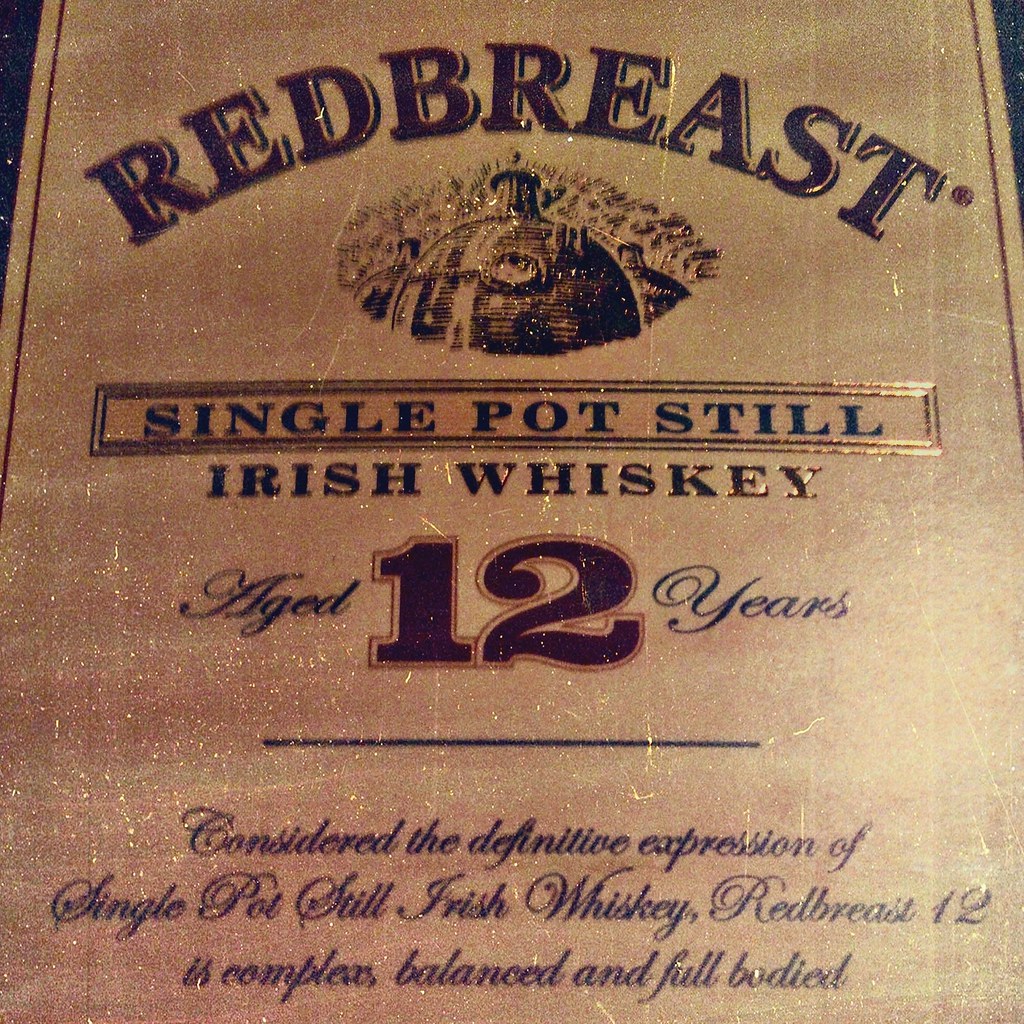This close-up photograph showcases the label of a whiskey bottle, specifically from Redbreast. The label has a textured, golden appearance that looks aged and slightly scratched, adding a sense of vintage charm. At the top of the label, in a curved, stylized font, it reads "Redbreast". Below this, there is a distinctive logo depicting a round building with a smokestack and additional structures in the background, evoking the traditional distillery imagery. The text "Single Pot Still" is prominently highlighted, followed by "Irish Whiskey" and "Aged 12 Years" with the number 12 in large, outlined figures. Beneath this, in elegant black cursive, it states, "Considered the definitive expression of Single Pot Still Irish Whiskey, Redbreast 12 is complex, balanced, and full-bodied." The overall presentation of the label, from its detailed text to its golden, worn look, accentuates the premium and storied nature of the whiskey within.